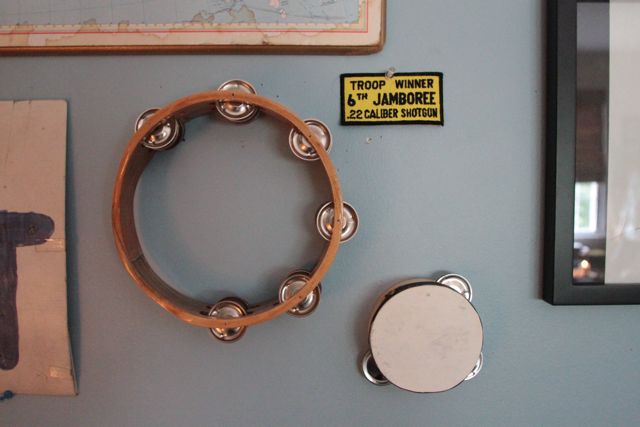The close-up image captures a section of a light blue painted wall adorned with an assortment of items. In the upper left corner, there is a framed picture with a brown, white, and pink border. Below this picture hangs a larger tambourine with a wooden frame, featuring six metal discs, though it appears to be missing some pieces. Next to it, partially obscuring the other frame, is a picture with a white background and a black letter that's difficult to discern. Toward the bottom right, a smaller tambourine is mounted on the wall, featuring only three metal discs. Above this smaller instrument is a rectangular piece of cloth that reads, "Troop Winner 6th Jamboree .22 caliber shotgun," featuring a yellow background outlined in black. A mirror is placed above this array, further enhancing the eclectic and detailed display on the wall.